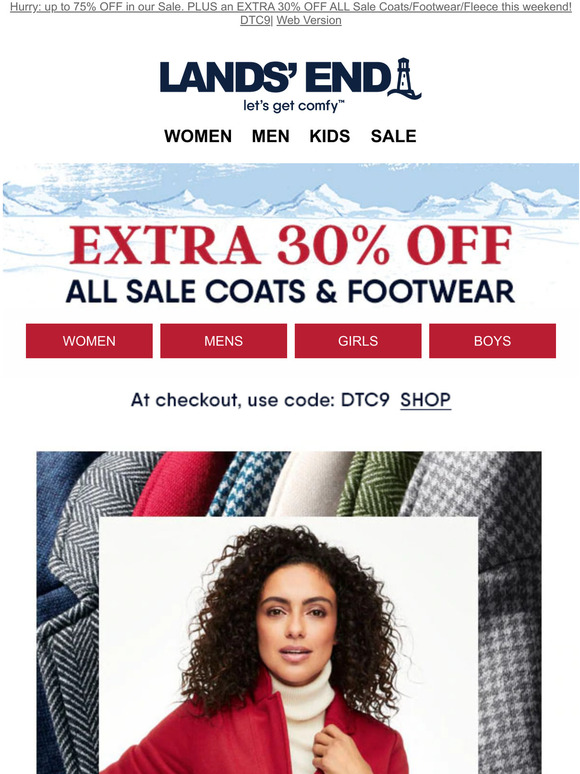This image is a promotional advertisement for Land's End, optimized for display on cell phones. At the very top, there is a blue underlined message that aims to capture attention with the offer: "Hurry! Up to 75% off in our sale plus an extra 30% off." This call-to-action encourages visitors to take advantage of the sale by visiting the website.

Below this promotional text, the Land's End website layout is depicted. The brand name "Land's End" is prominently displayed in large, bold blue font, accompanied by their signature lighthouse logo, symbolizing a coastal theme. The company's slogan, "Let's get comfy," is positioned right underneath the logo, reflecting their focus on comfortable clothing.

The advertisement features four main drop-down menu options: Women, Men, Kids, and Sale, providing easy navigation for shoppers. Beneath these menus, there is a prominent banner ad that highlights an additional discount. In bold red font, it announces "Extra 30% off," and in bold black font, it specifies that this discount applies to "All sale coats and footwear." The ad also includes information on the promotional code to be used at checkout to avail of these discounts, thus encouraging immediate action from potential customers.